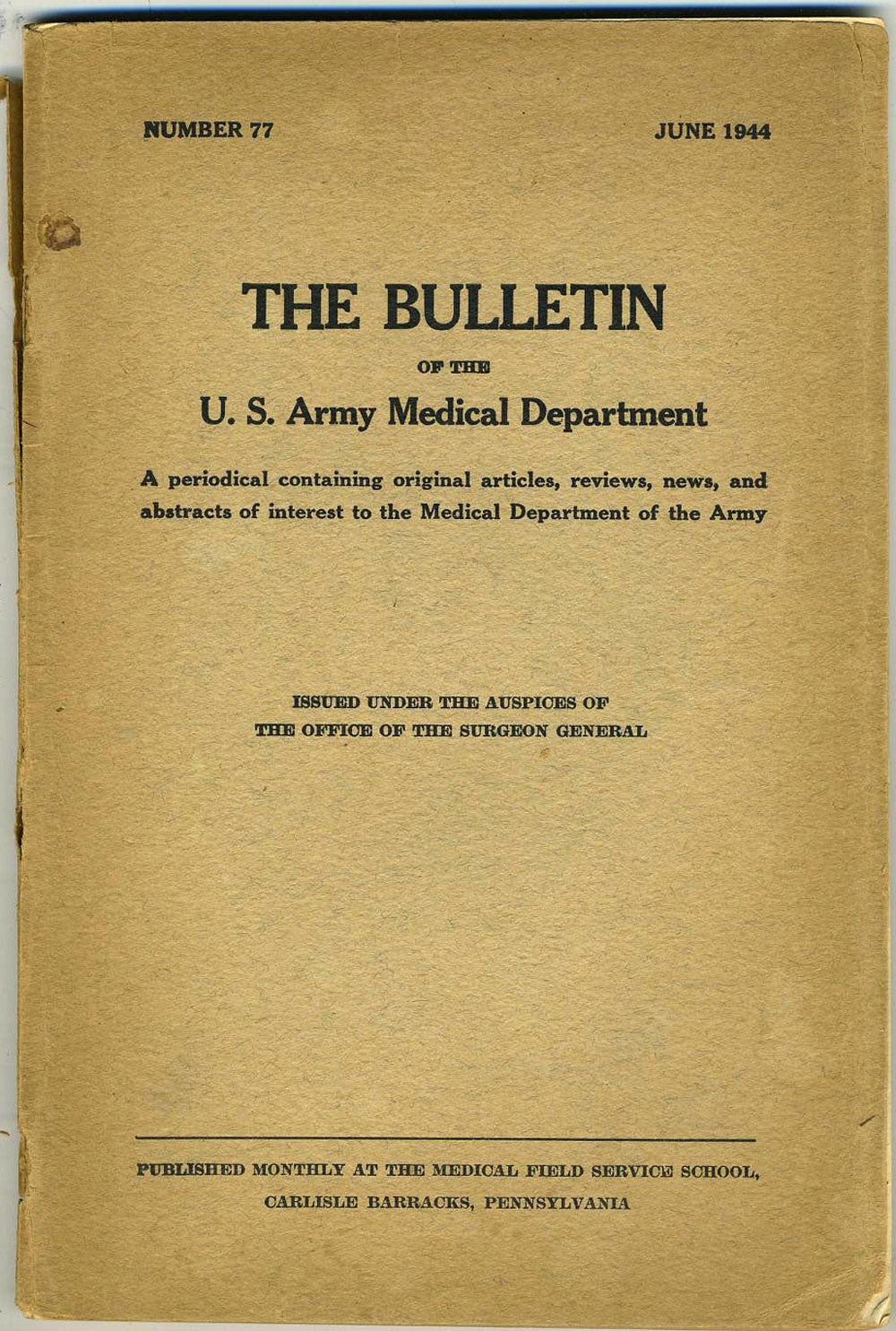This image depicts an aged and yellowed title page from the Bulletin of the U.S. Army Medical Department, dated June 1944 and designated as number 77. The page has a worn, brown cover with black text. At the top left, it states "Number 77," and on the right, "June 1944." Centrally, it prominently reads "Bulletin of the U.S. Army Medical Department," followed by a descriptor: "A periodical containing original articles, reviews, news, and abstracts of interest to the Medical Department of the Army." Midway down, it is noted as "Issued under the auspices of the Office of the Surgeon General." At the bottom, it specifies: "Published monthly at the Medical Field Service School, Carlisle Barracks, Pennsylvania." The document shows signs of wear, indicating its historical significance, with minor indentations and some damage suggesting it's beginning to fall apart. The image has a vague white-gray border, emphasizing that this is clearly a scan or photo of an old document.